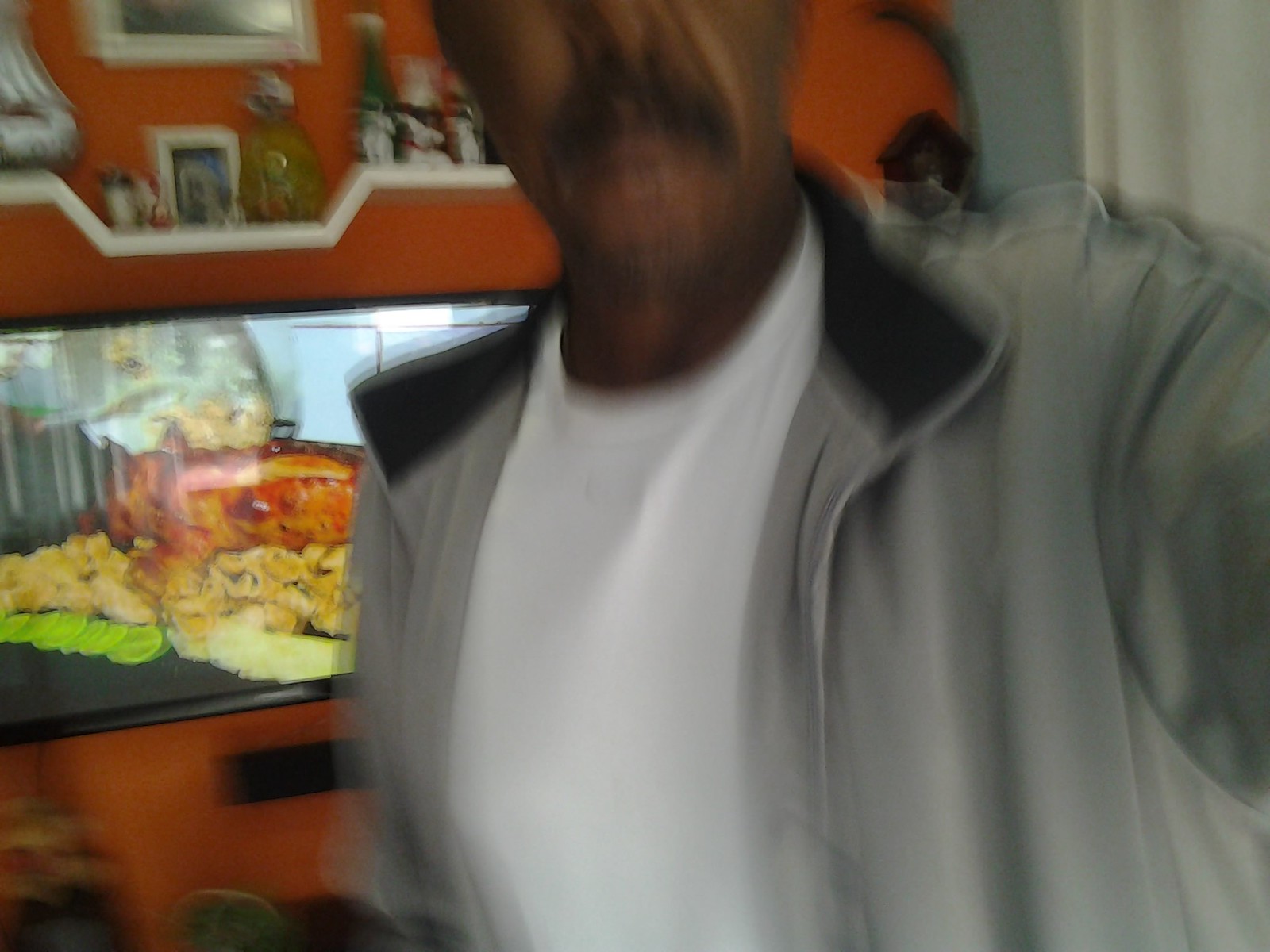The image depicts a tan-skinned man with a thick black mustache, wearing a white T-shirt beneath an unzipped gray jacket with a black collar. He is facing the camera for a selfie, but the photo is quite blurry, particularly on the left side. In the background, an orange wall features a white shelf. On the shelf, there is a white picture frame, possibly holding a silver or white vase, and green and yellow bottles. Above the shelf, there's a white-framed picture that partially appears above a black-framed painting, which might depict a cooked pig. On the right side of the image, there are flowy white curtains, which are only visible from the top part. The scene also includes what looks like an outer area of a television screen, displaying a scene with various vegetables in its background.